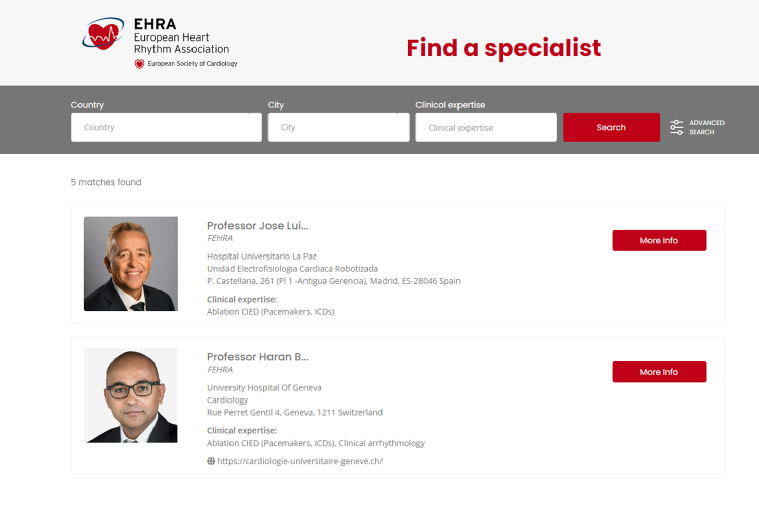This image showcases the European Heart Rhythm Association (EHRA) website interface. At the top, the menu bar features a heart icon accompanied by a static line, followed by "EHRA" in bold black text. Directly beneath this, the full name "European Heart Rhythm Association" is displayed in black. Adjacent to this, there is another logo with a heart representing the "European Society of Cardiology."

To the right, in red text, it reads "Find a Specialist." Below this heading, there is a dark gray box labeled "Country" with an accompanying white text box for user input. Next to it, a similar setup exists for "City," both labels in white. Further to the right, there is a "Clinical Expertise" label and a corresponding text box for users to specify their needs. Lastly, there's a red search bar with white font and an adjacent filter icon labeled "Advanced Search."

Below the search section, the website displays a result of "5 matches found." The first two listings are partially visible. The first entry features Professor Jose Luis, affiliated with Hospital Universitario La Paz in the Unidad Electrofisiologica Cardiaca Robotizada. His clinical expertise includes Abhiaton, CIEO, Pacemakers, and ICDs. To the right of this entry, there's a red "More Info" button with white text. A photograph of Professor Jose Luis appears on the left side of his entry.

The second entry features Professor Haran B, with his detailed designation as FEHRA at the University Hospital Geneva Cardiology Department. This listing also includes a red "More Info" button with a white font and a picture of Professor Haran B below the text.

This detailed description provides a comprehensive overview of the EHRA website’s layout and user-interface features.